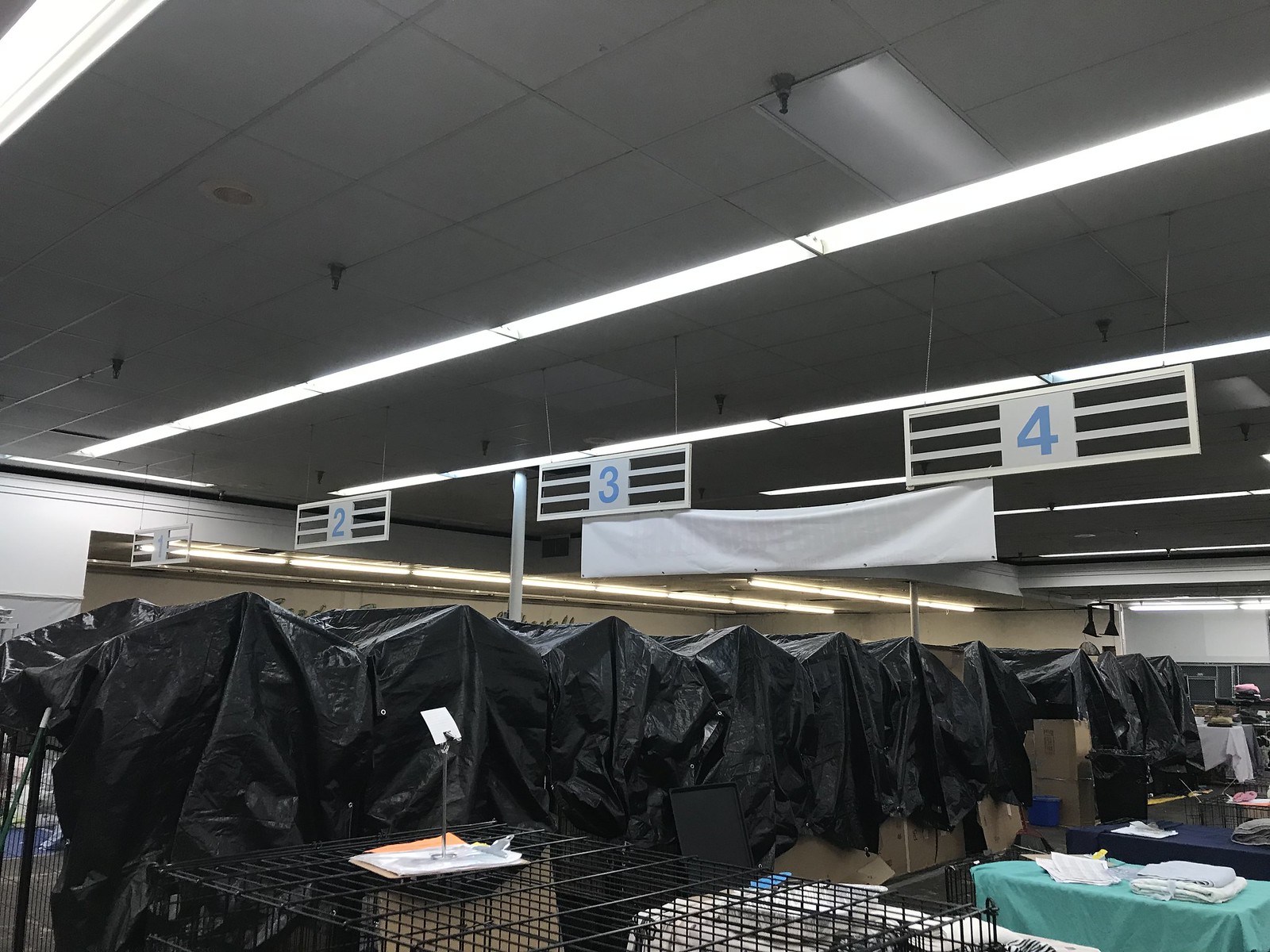The image depicts the interior of a manufacturing facility, captured in a horizontal layout. The facility is characterized by its high drop ceiling adorned with long rows of fluorescent lights, providing bright illumination throughout the space. Below, there are systematic rows of triangular-topped items covered in black tarps, extending diagonally from the lower left to the upper right of the image. 

Wire table cages filled with various items are strategically positioned within the facility. Some tables display folded cloths, while others have manila envelopes and a clipboard atop them, suggesting organized storage or workstations.

Suspended from the ceiling, rectangular metal signs with blue numbers on a white background denote the rows of the black-covered items, aiding in navigation or identification. Row one is situated in the furthest distance towards the back on the center left, and row four is the closest, positioned in the upper center right of the frame. The orderly arrangement of equipment and the methodical layout underscore the facility's industrial precision and organization.